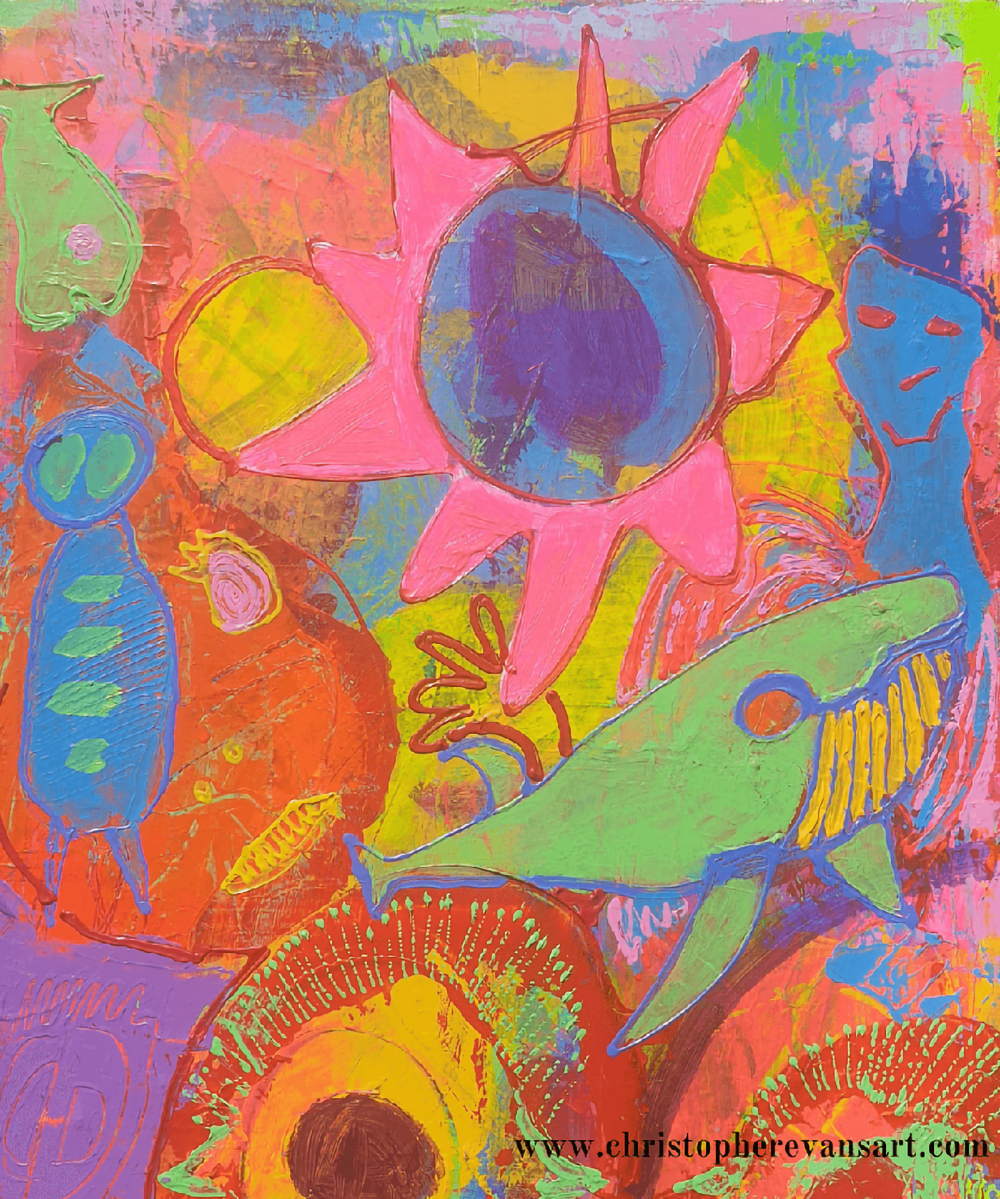The painting is a vivid and colorful abstract composition, showcasing a vibrant palette of neon pinks, greens, oranges, yellows, blues, purples, and reds. The central focus appears to be a sun or an eye, adorned with pink spikes and a blue and purple center, emanating blue rays. Below this, there is a whimsical green creature resembling a shark or a whale with big yellow teeth, a yellow chin, and one orange and one black eye. To the left, a blue, childlike figure with oversized green eyes and green buttons is holding itself, appearing as though it has an ant-like body. Nearby, above it, floats a green fish with a pink eye that is oriented upside-down.

On the right side, there's a blue figure reminiscent of a bowling pin with eyes, adding to the quirky, juvenile feel of the artwork. Additionally, a yellow avocado with peacock feathers is depicted at the bottom. Several other abstract forms, such as an orange gourd-like shape and what might be considered a tree or a blob with a yellow face, further populate the scene. Bright splashes of colors add to the chaotic and playful composition, evoking a sense of a child's imagination and creativity. The painting has the artist's website, www.ChristopherEvansArt.com, prominently displayed in the bottom right-hand corner.